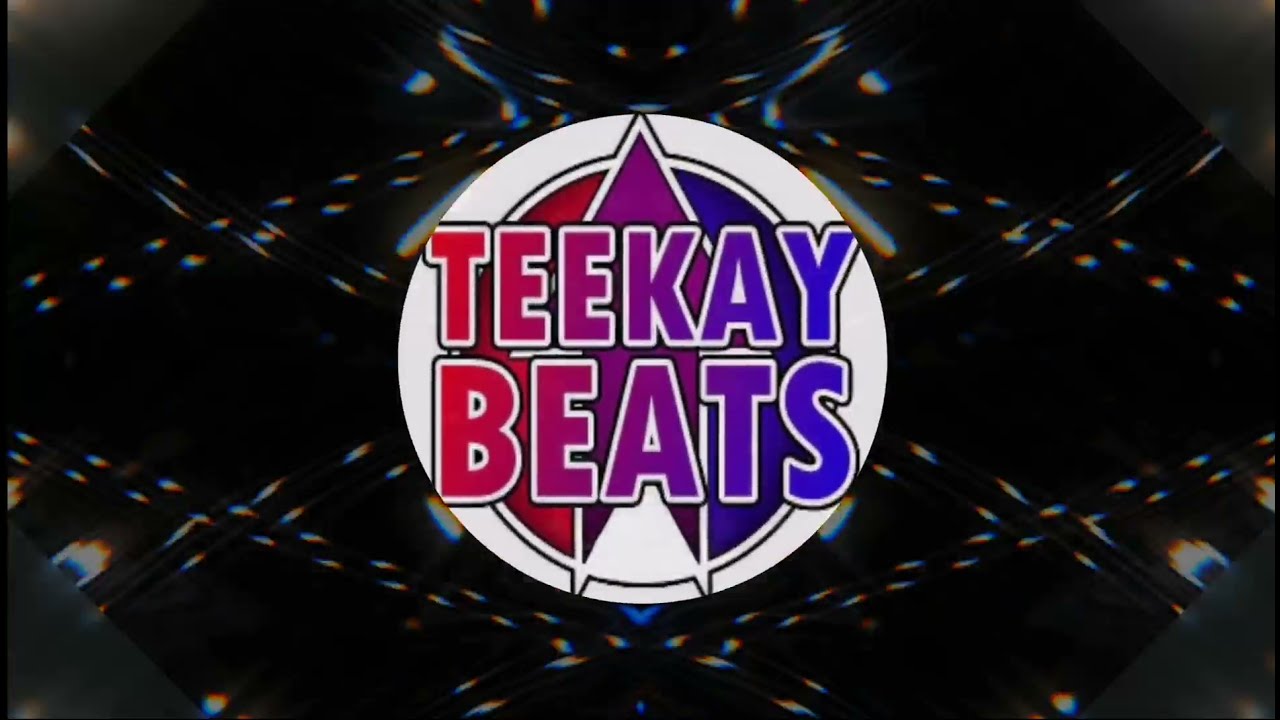The image is a graphical design with a black background, accented by light gray corners cut in triangular shapes. Emerging from these corners are beams of red, white, and blue light forming a vibrant frame around the centerpiece. At the center of the design is a white circle, inside of which lies a diamond pattern composed of interconnected chain links, reflecting a spectrum of colors from blue to red. Encircled within this white disc, the title "T-K-Beats" is prominently displayed in bubble letters. The text showcases a gradient effect, transitioning smoothly from red on the left, through pink and purples in the middle, to royal blue on the right.